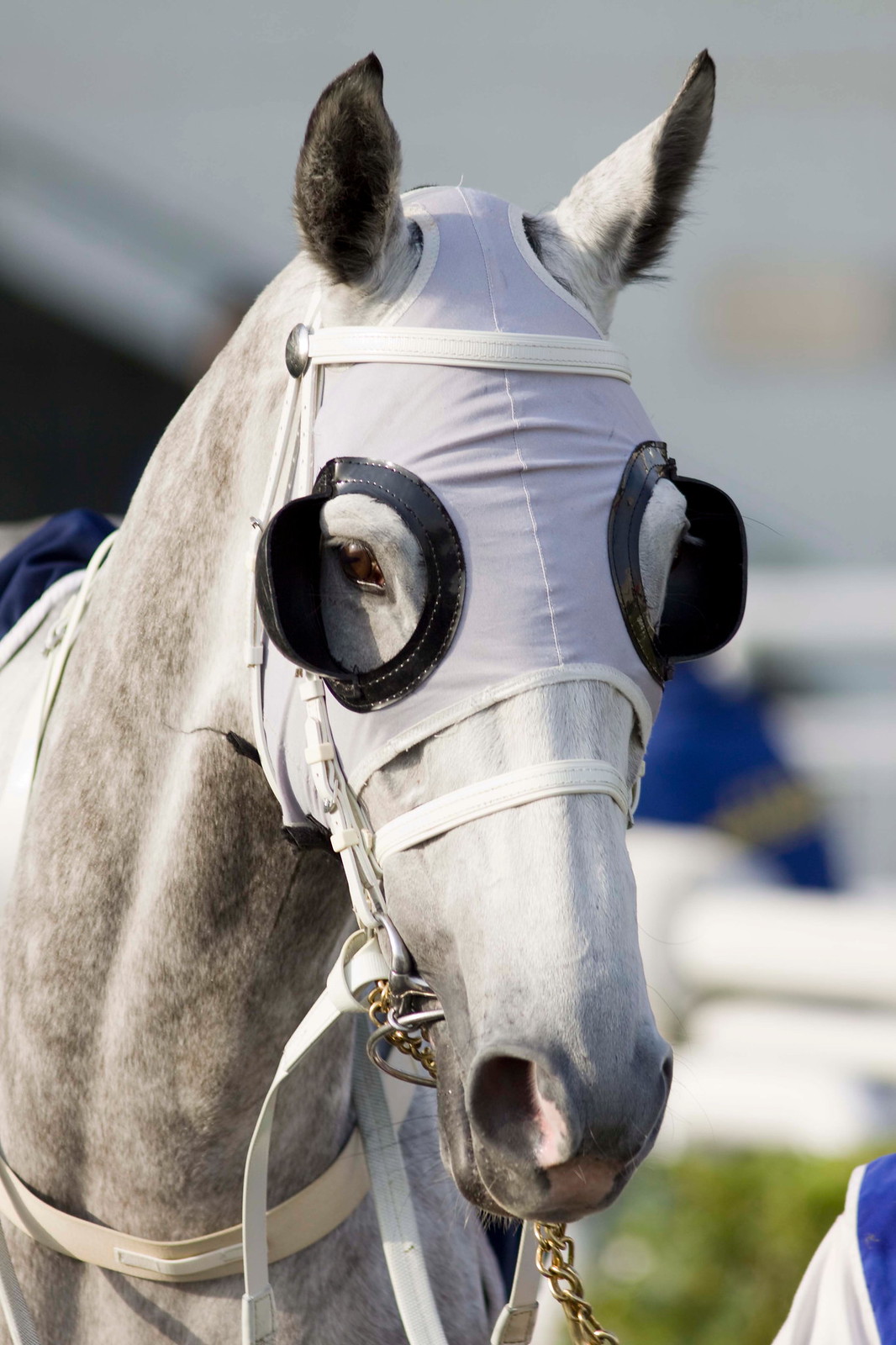The photograph is a professional, close-up image of a racehorse, likely during a race. The horse is predominantly white with grey shading around its nose and brown shading along its neck. The background is blurred, showing the light grey daytime sky, a bit of white fencing, and some greenery. There is also a blue object that appears to be the arm of a person, possibly a jockey, and a glimpse of a blue jersey in the bottom right corner. The horse wears a light purple mask that somewhat resembles a pair of underpants, with black-rimmed open eye covers and attached blinders. A small gold chain hangs from its neck, and the mask extends along the horse's back with a slight bit of blue visible. The horse is looking slightly to the right, just away from the camera.